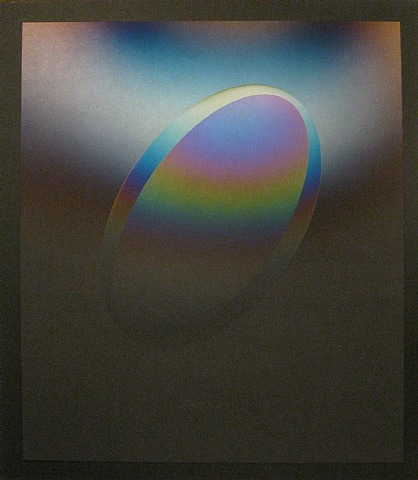The image is an abstract, almost painting-like illustration featuring a central, slanted zero or oval against a gradient background ranging from black at the bottom, transitioning through dark blue, and finally to white at the top. Surrounding the entire image is a dark gray or black border, creating a frame for the primary subject. The zero shape in the center mirrors the background gradient but is turned slightly to the right. Its gradient transitions from dark blue to white, with a glossy metallic sheen suggesting a light glare at the top. Within this zero shape lies another gradient, inverted compared to the outer one, showcasing a vibrant spectrum of colors—gray at the bottom, progressing through red, blue, green, yellow, and other hues in an unconventional rainbow sequence. The overall effect is a striking, chromatic, and metallic composition with layers of gradients providing depth and visual interest.